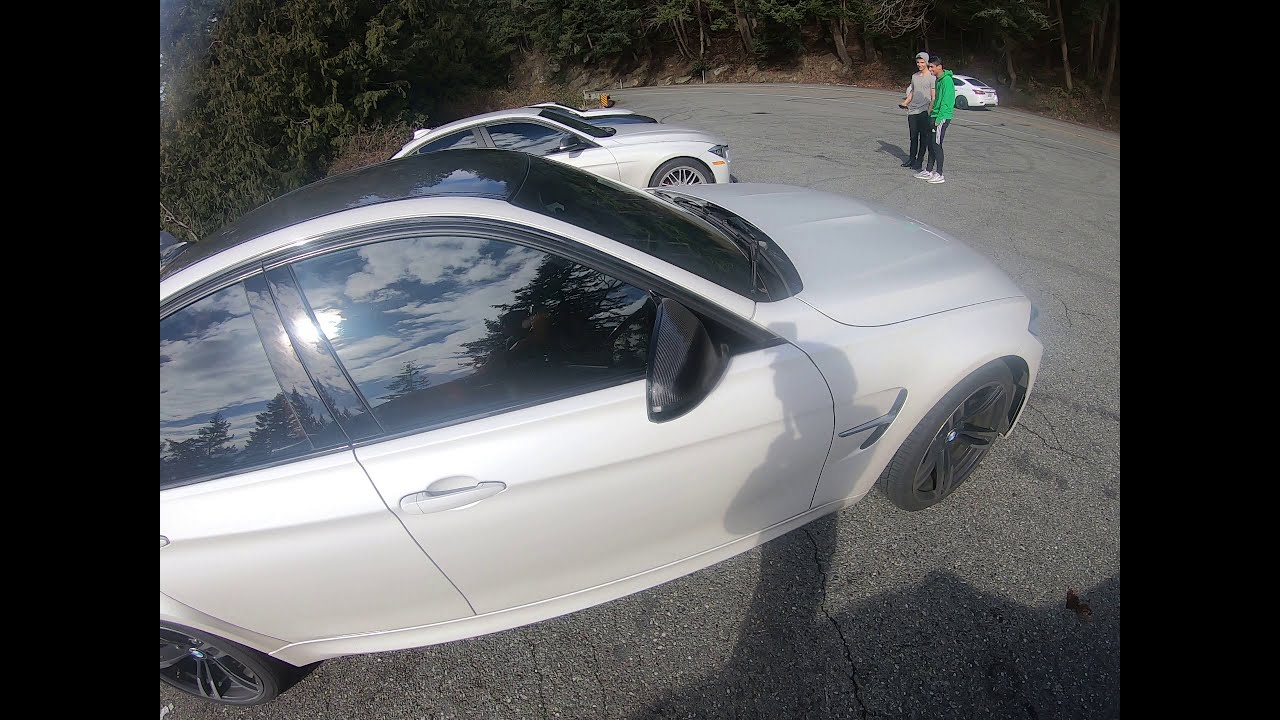The photograph captures an outdoor parking lot scene with a semi-circle road in the background, flanked by thin trees with brown trunks on both sides. The parking lot is filled with primarily white, expensive-looking sports cars, including one prominently-placed BMW. A single black car stands in contrast amongst them. Two young men, one in a green hoodie and the other in a gray shirt with a backwards hat, both wearing black pants and sneakers, are engaging in conversation while gazing at the cars. The sun casts visible shadows, including that of the photographer, onto the vehicles and the ground, which consists of clumps of dirt with scattered greenery. To the right, a white car is moving along the curved road. The photo is framed by black rectangles on the left and right, adding a touch of compositional balance.